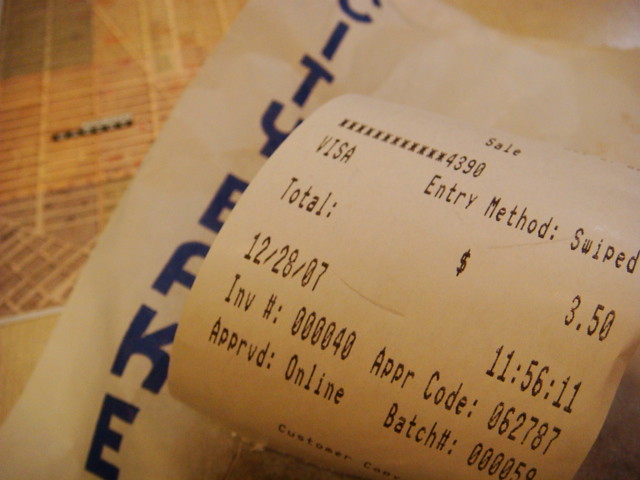The image depicts a close-up shot of a small, square-shaped receipt paper that is slightly curved. The receipt, processed via a Visa card swipe, bears the date "12-28-07" and the time "11:56:11 seconds." At the bottom of the receipt, the text "Customer Care" is clearly visible. This receipt is positioned atop a white bag with blue writing that reads "City Bake" in a distinct blue font. The bag rests on a table featuring a pattern of squares and rectangles, colored in various shades of light yellow.